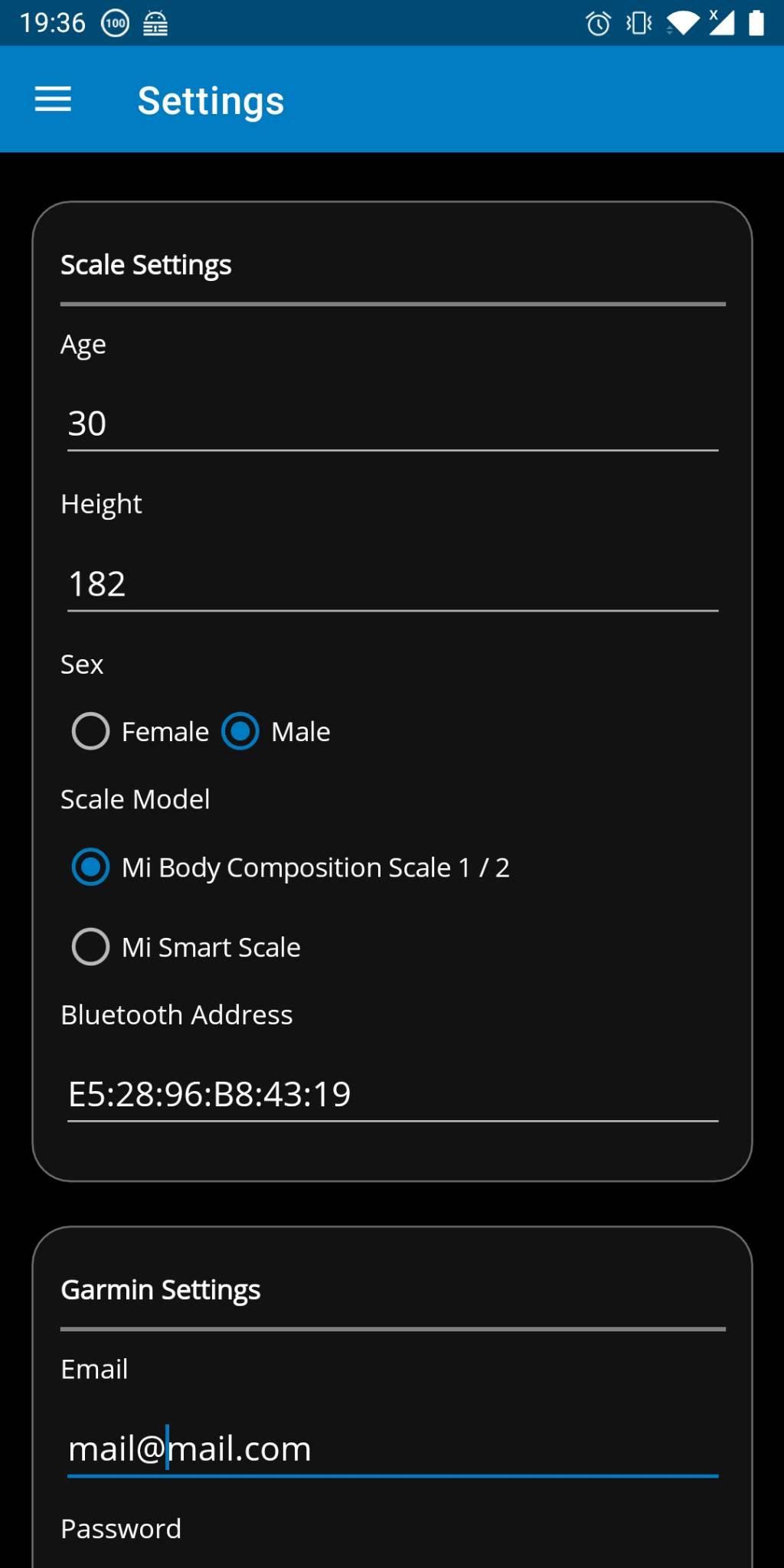This is a detailed snapshot of a smartphone screen with a black background. At the top, the status bar displays the time as 19:36, along with several icons including a lock, an alarm clock, a vibrate symbol, Wi-Fi signal, signal strength, and a nearly full battery percentage. Below the status bar, a small blue banner contains the word "Settings" written in white text. The rest of the page continues in white text on a black background.

Directly beneath the blue banner are three white horizontal lines that may represent a menu icon. Following that, there is a section titled "Scale Settings." This section details user metrics: age is set to 30, height to 182, and gender is selectable via radio buttons for female and male, with the male option currently selected. The selected scale model is "High-Body Composition Scale 1.5," alongside another, unselected option labeled "MI Smart Scale."

Further information includes a Bluetooth address listed as E5.28.96.BA.43.19. Below that, there's a section titled "Garmin Settings," showing an email address "mail at mail.com." Finally, at the bottom of the screen, there is a field labeled "Password."

Overall, the screen's primary color scheme is white text on a black background, with the most prominent color being the blue banner at the top signifying the settings menu.